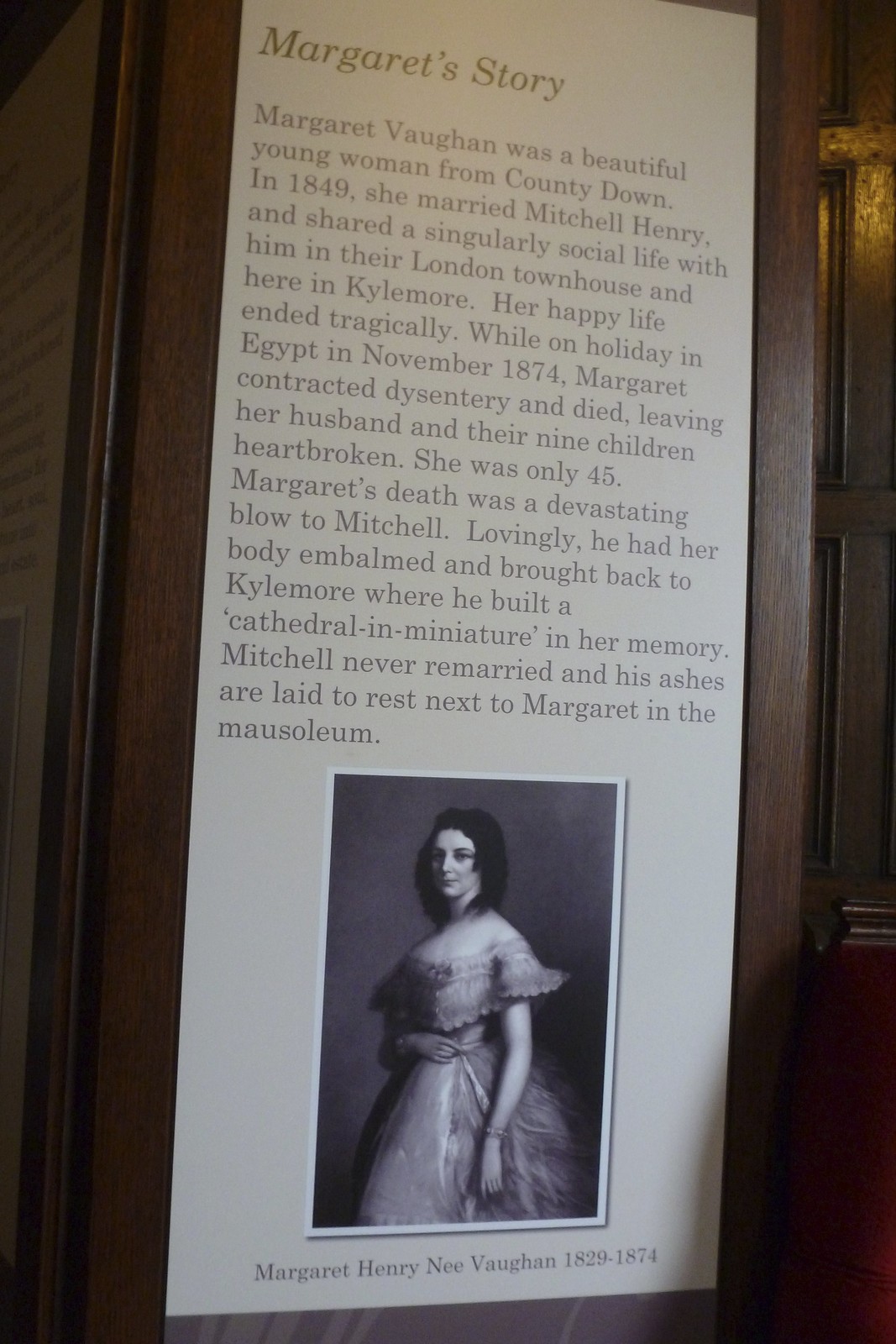The photograph depicts a well-crafted sign mounted on a beautiful wooden wall, likely situated in a museum or historic site. The sign, bordered in wood, is beige with brown lettering and is titled "Margaret's Story." At the bottom of the sign, a black and white image of a woman in a stunning historical ball gown is displayed, captioned "Margaret Henry née Vaughan, 1829-1874." 

The text on the sign narrates the poignant tale of Margaret Vaughan, a beautiful young woman hailing from County Down. In 1849, she married Mitchell Henry and enjoyed a socially vibrant life with him both in their London townhouse and in Kylemore. Unfortunately, her life was cut short while on holiday in Egypt in November 1874, where she contracted dysentery and passed away at just 45 years old, leaving behind her heartbroken husband and nine children.

Mitchell Henry was profoundly affected by Margaret's death and took great care to have her body embalmed and transported back to Kylemore. In her loving memory, he constructed a miniature cathedral. Mitchell never remarried and, upon his death, his ashes were laid to rest beside Margaret in the mausoleum, eternally united in love and memory.